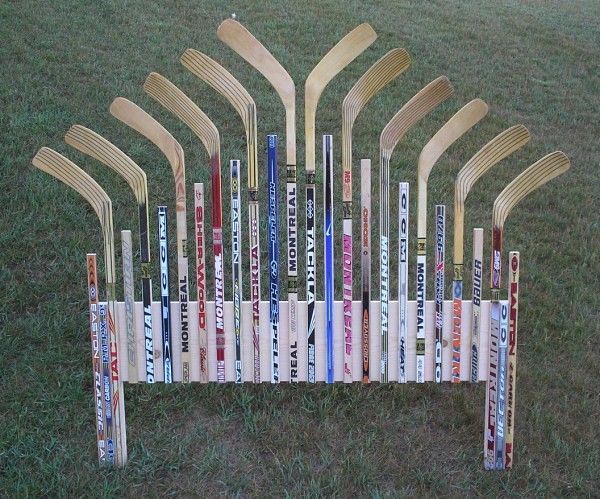In the center of the image stands an intricate sculpture made from numerous hockey sticks, meticulously arranged into a visually striking, symmetrical pattern. The sticks, each displaying unique designs, labels, and vibrant team colors, are chopped into halves. The intact, colored ends of these 24 sticks are aligned in an inverted V formation, while the cut segments without the blade portion fill the gaps to enhance the structure's sense of spacing and balance. The sticks are mounted on a light beige wooden platform, with the grain of the wood running horizontally across the base, forming a house-like shape with a hollow rectangle at the bottom supported by two vertical poles on either side. This artistic installation, set against a backdrop of a slightly dry, green field hinting at early fall conditions, captures the eye with its thoughtful organization and unique blend of elements, standing prominently in the middle of the outdoor scene.